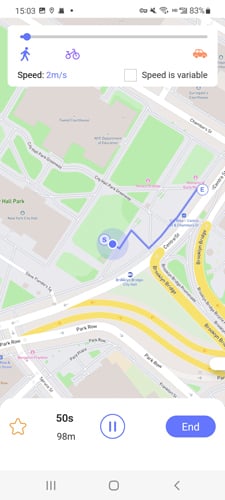The image features a digital map interface, likely from a navigation app. The upper section of the interface includes a horizontal progress bar, which is minimally filled with a blue line, possibly indicating the journey's progress. To the right of the progress bar, there are three icons in sequence: a walking figure, a bicycle, and an orange car, suggesting different modes of transportation.

In the middle portion of the map, a route is clearly marked, showing the path the user needs to follow. Alongside this, a section displays the current speed in meters per second (m/s), with the speed value dynamically changing.

At the bottom of the interface, there is a prominent button labeled "End," likely used to conclude the navigation session.